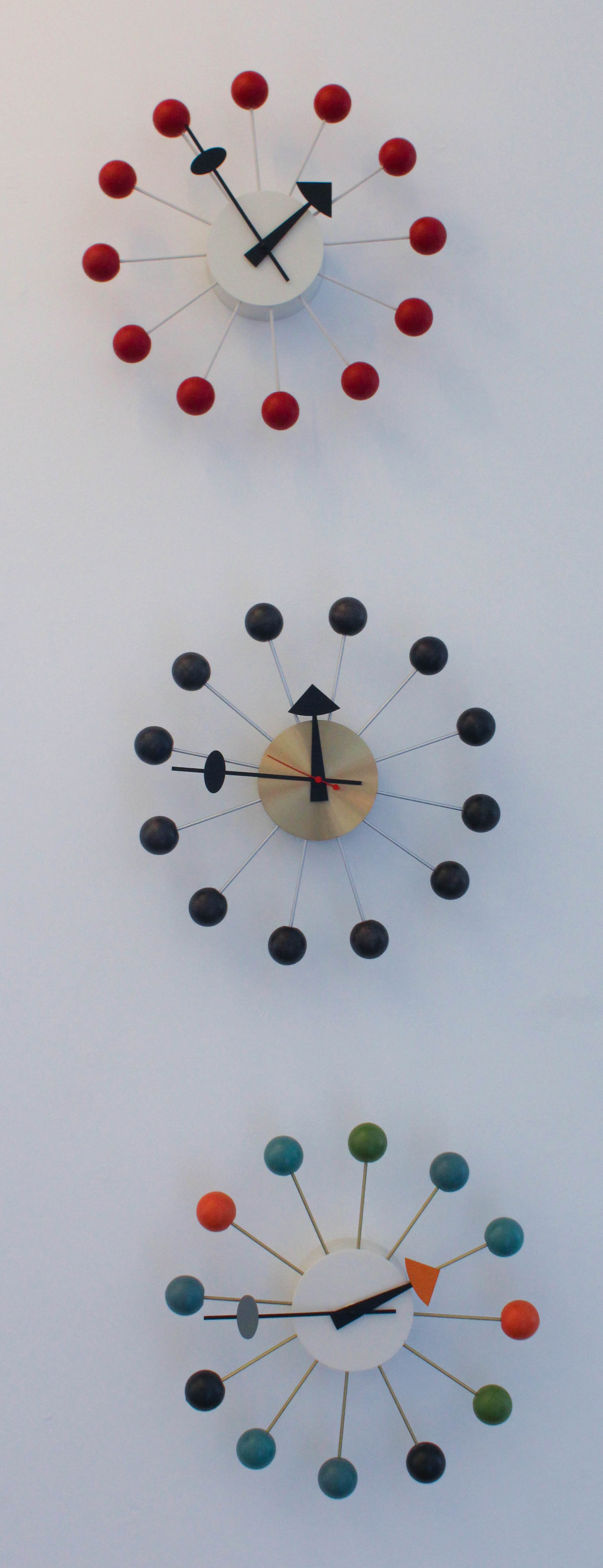This is a crisply detailed photograph featuring three abstract clocks mounted on a pristine white wall. The first clock has a minimalist design with a white clock face, black hands, and is adorned with red circles. Its hands are delicate and silver, adding an elegant touch. The second clock stands out with its deep navy hue and bronzy clock face. It has black hands and a striking red second hand, with navy circles embellishing the face. The third clock displays a playful design featuring a white clock face and black hands, one of which has an orange triangle marker. The face is decorated with multicolored round balls in shades of orange, blue, green, and black. The image is exceptionally clear, showcasing subtle shadowing effects on the white wall, with no other objects present to distract from the unique timepieces.